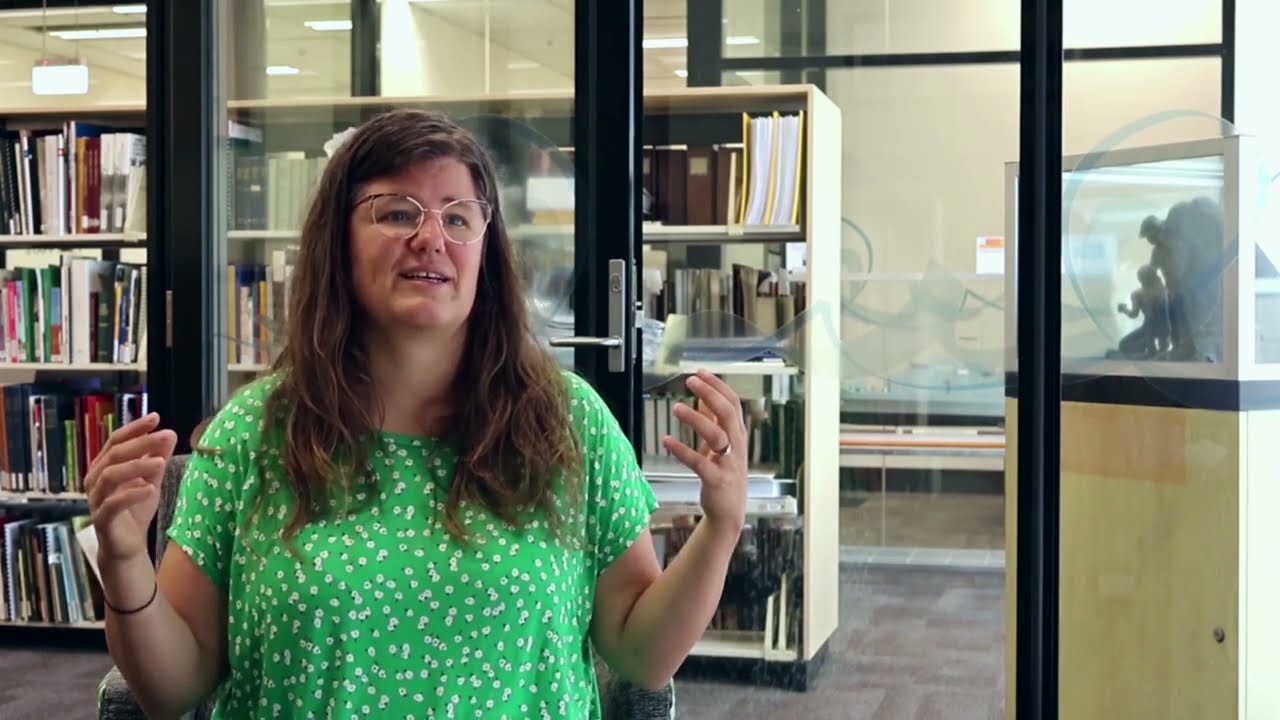In the image, a middle-aged, heavy-set Caucasian woman is featured prominently. She is wearing a green, short-sleeved polka-dotted dress and has light brown, wavy hair that falls just below her shoulders. She also sports thin wire-rimmed glasses. The woman is standing inside a well-lit library, in front of a glass door with black metal frames. Her posture and expression suggest she is animatedly explaining something, with her hands raised and bent at the elbows. She seems to be talking to someone off-camera on her right, hinting at an engaging conversation. Behind her, tall bookshelves filled with books and folders emphasize the academic setting. A white bookshelf and a display case with a statue are also visible through the glass door, adding to the scholarly ambiance. To the far back, there appears to be a picture or a lamp and a table, although the exact details are not clear. The woman appears happy and enthusiastic as she interacts, potentially indicating that she is involved in an interview or a similar activity.